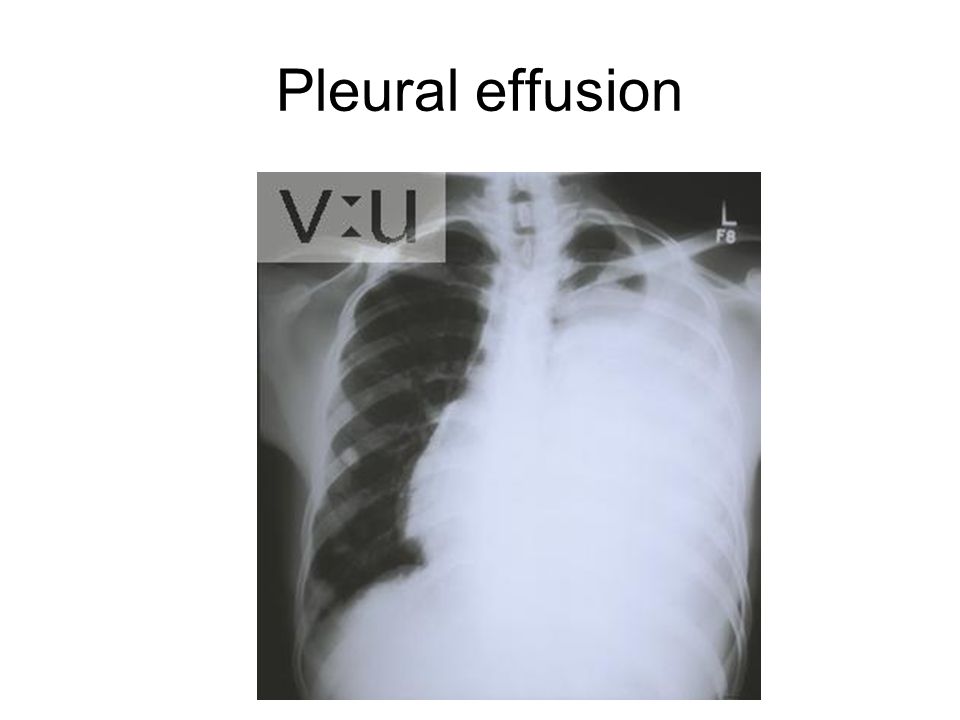The image depicts a detailed chest x-ray of a person, labeled at the top in black letters as "Pleural Effusion." The x-ray itself occupies a square shape beneath this label. The upper left-hand corner of the x-ray features black text within a light grey rectangular box, marked with the letters "V" and "U," with an upside-down triangle and a right-side-up triangle between them. The main portion of the x-ray shows the rib cage prominently illuminated in white, contrasting sharply against the black background. The left side of the chest appears clear with a dark background indicating an area where the lung should be, while the center and right side of the chest are predominantly white, indicating a pleural effusion. In the upper right-hand corner of the x-ray, there is a white letter "L" with "F8" positioned below it.